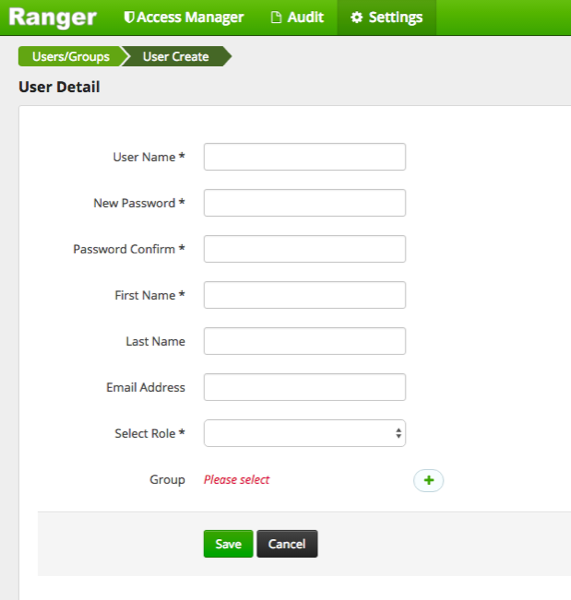This image is a detailed screenshot of a login page for the Ranger Access Manager. The layout is in a square format with a green banner stretching across the top. On the upper left corner of the banner, "Ranger" is prominently displayed in white text, accompanied by a shield icon. Adjacent to the shield icon, the words "Access Manager" are visible. Directly to the right of this, there is a paper icon followed by the label "Audit." Next to "Audit," there is a darker green section featuring a widget icon and the word "Settings."

Below this main banner, there is a green rectangular shape with a pointed end on the right, centrally labeled "User / Groups." This is followed by another rectangular shape, slightly darker in green, also with a pointed right end, labeled "User Create." The label "User Detail" is placed below these rectangular shapes.

Further down, there are seven vertically aligned text fields categorized for: Username, New Password, Password Confirm, First Name, Last Name, Email Address, and Select Role. Below these fields, the term "Group" appears with a dropdown menu prompt "Please Select." Centered at the bottom of the page, two prominent buttons labeled "Save" and "Cancel" are situated, providing final action options for the user.